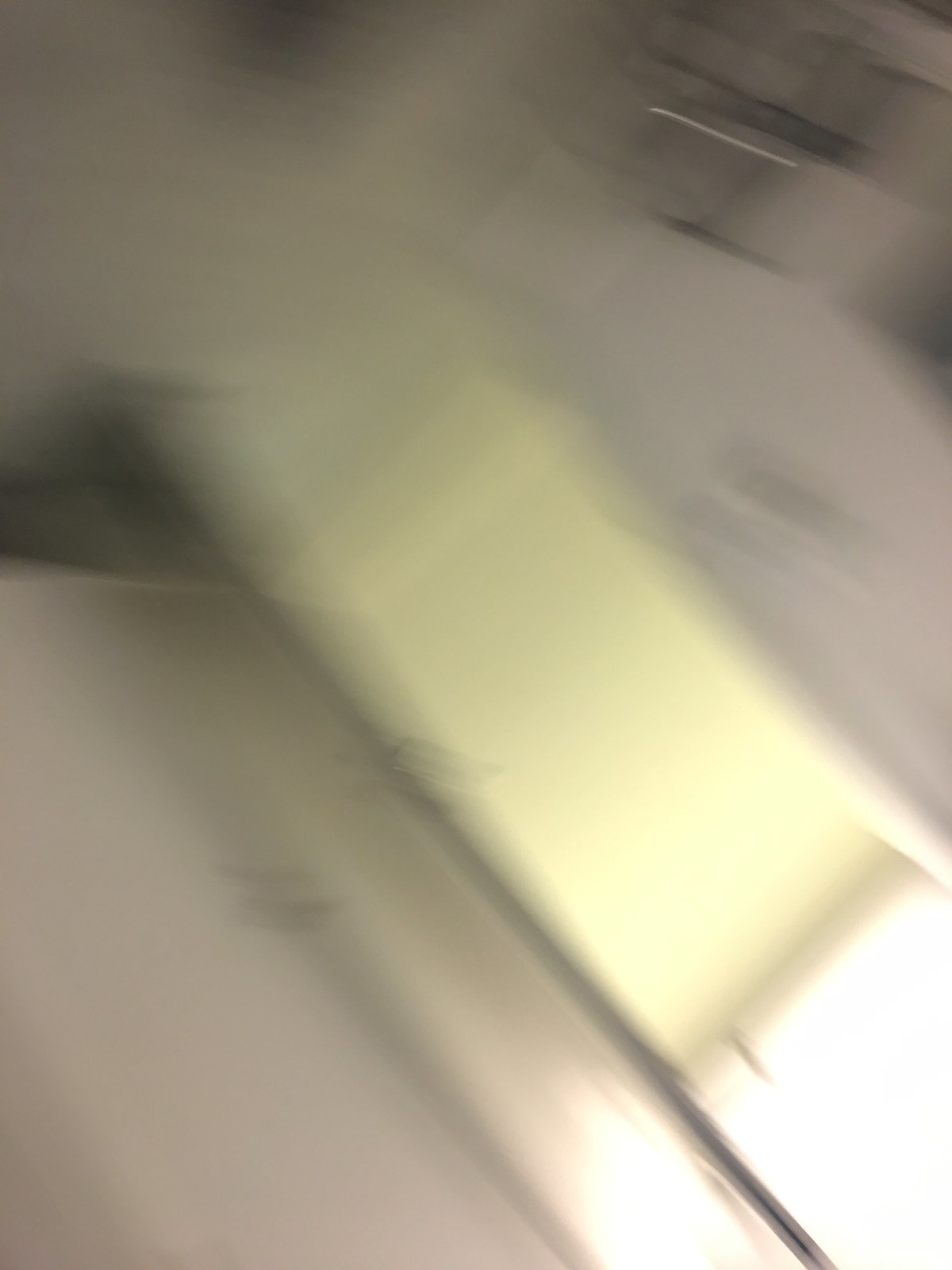The image is an extremely blurred photograph that appears to have been taken upside down, making it challenging to distinguish specific details. The primary focus seems to be an open doorway through which a tan-colored room is visible. The image is dominated by dull white colors on either side of the doorway. In the upper right-hand corner, there is a silver object potentially resembling a mesh wire basket or shopping cart mounted on a white wall. Adjacent to the doorway, towards the bottom left of the photograph, a light source is emitting a bright reflection across the wall. There also appears to be a cabinet with handles on the right side and a rectangular shape that possibly resembles a window shade that is partially drawn up, allowing light to filter through. Despite the heavy blurriness, there may be a paper with writing attached to a wall in the background.